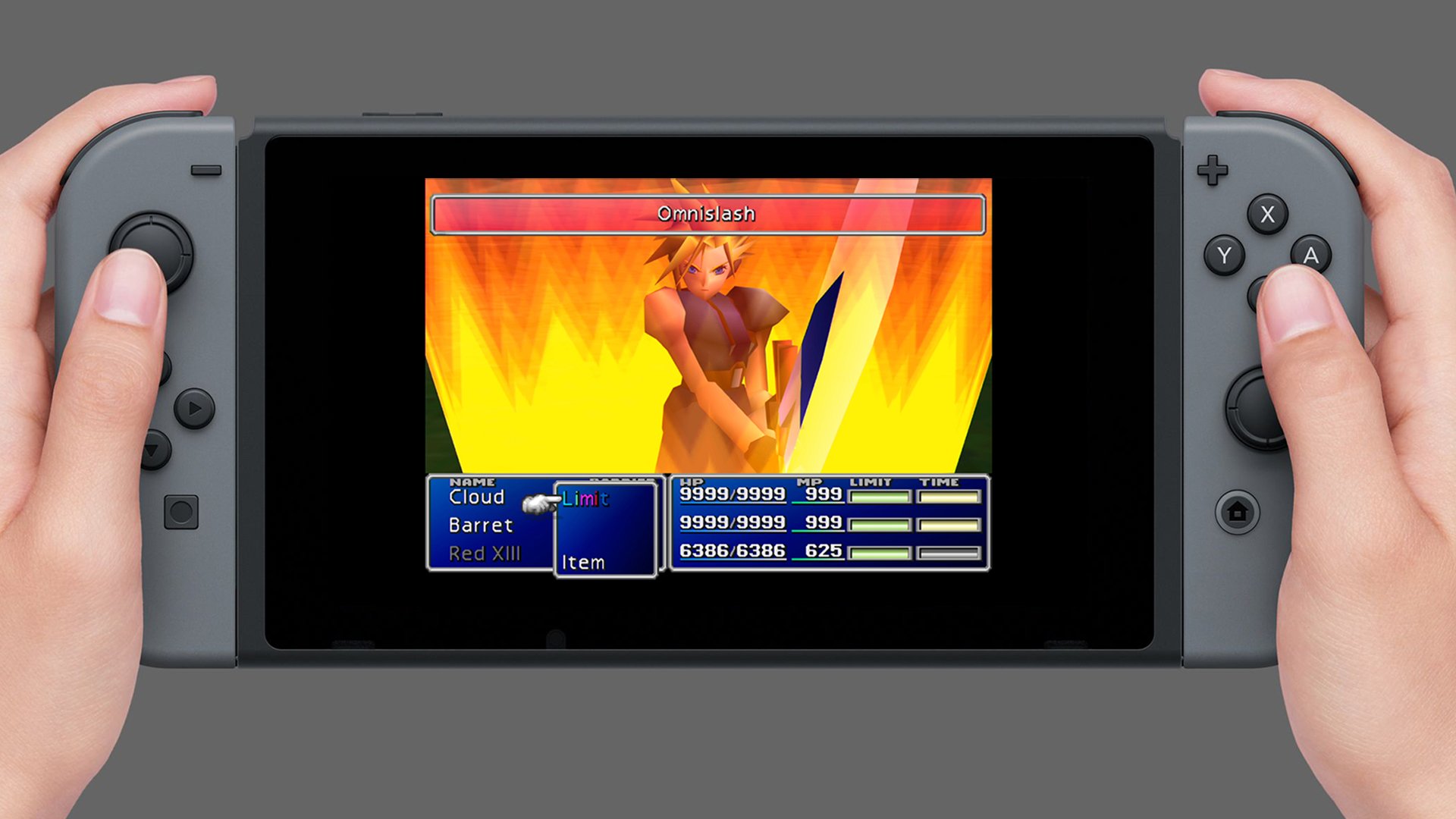The image depicts a person holding a gray Nintendo Switch, with both hands gripping the gray Joy-Con controllers on either side of the device. The Joy-Cons feature black buttons, with white letters on the right-hand side buttons labeled X, Y, and A. A thumb rests on another button near the home button below the joystick on the right controller. The left controller's joystick is positioned at the top, with arrow buttons located beneath it, and the top of the left joystick shows a minus symbol, while the top of the right joystick shows a plus symbol. 

The central focus is the Nintendo Switch’s screen, which has a significant black border around it. On the screen, there is a vivid and dynamic scene involving a character with spiky blonde hair. This character, likely from the game "Final Fantasy," is enveloped in flames that transition from yellow to red, indicating the intensity of the action. The character seems to be performing an attack, identified by the word "Omni Slash" displayed alongside a red bar at the top. There is also a mystical, blue shape in the background, adding depth to the scene. Below this, an in-game interface appears featuring a scoreboard with blue blocks containing white text and green bars, and the names "Cloud" and "Barrett" are visible on the screen.